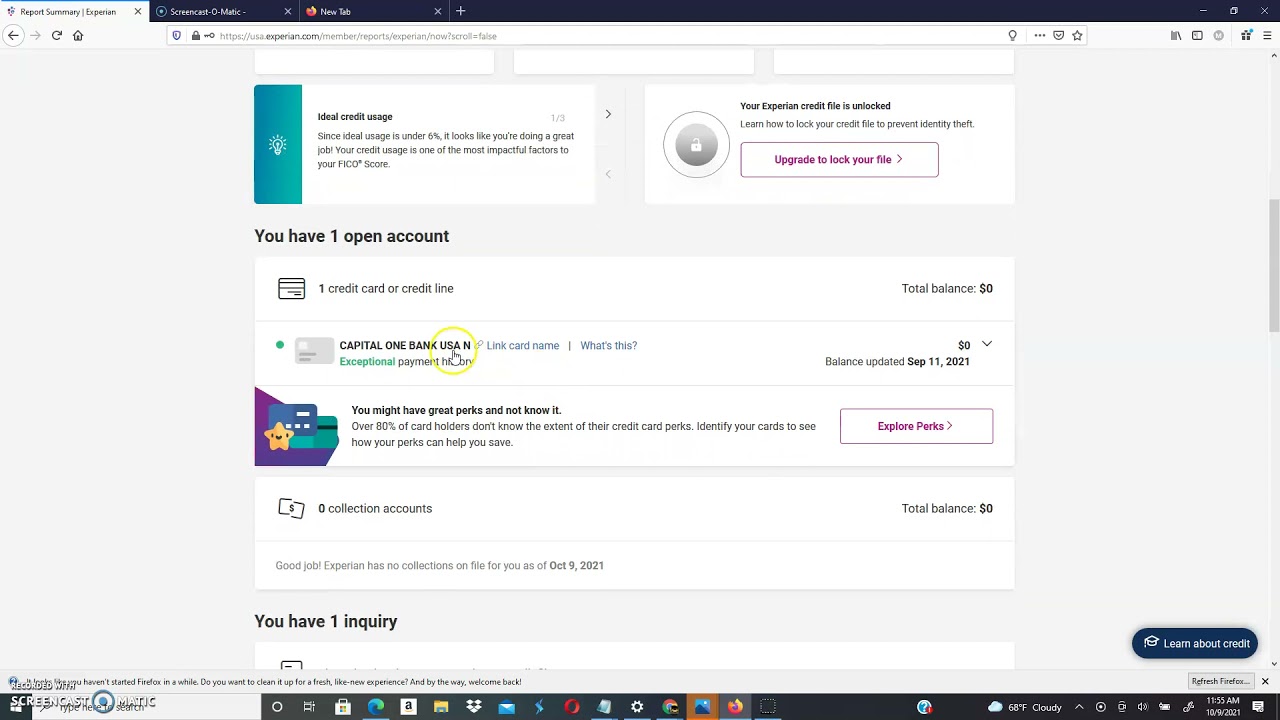This image, presented in portrait orientation though captured in landscape mode, showcases a Firefox browser window with three open tabs. The primary tab being viewed is titled "Report Summary Experience," while the secondary tabs are "Screencast-O-Matic" and "New Tab." A visible Screencast-O-Matic watermark confirms the recording tool is active, positioned at the bottom left of the screen.

In the bottom right corner, the system clock displays a time of 11:55 a.m. with a date stamp of October 9, 2021. Various icons populate the taskbar at the bottom of the screen, indicating numerous active applications or notifications.

The main section of the screenshot features an Experian credit report summary. At the top, a highlighted section about "Ideal Credit Usage" is visible, indicating the user's Experian credit file is currently unlocked. A red notification suggests upgrading to lock the file for added security.

Following that, the summary details the user's credit status: 

- **Open Accounts:** One 
- **Credit Cards/Credit Lines:** One 
- **Total Balance:** $0

A specific entry for "Capital One Bank USA" is emphasized, marked with a yellow circle around it and the user's cursor positioned over it. This entry notes an "Exceptional Payment History" with a balance of zero dollars, last updated on September 11th.

Further down, a row indicates a promotional message about potentially undiscovered perks, accompanied by a purple "Explore Perks" button on the right. Additional details confirm zero collection accounts and a total balance of zero, with a highlighted note indicating one recent inquiry.